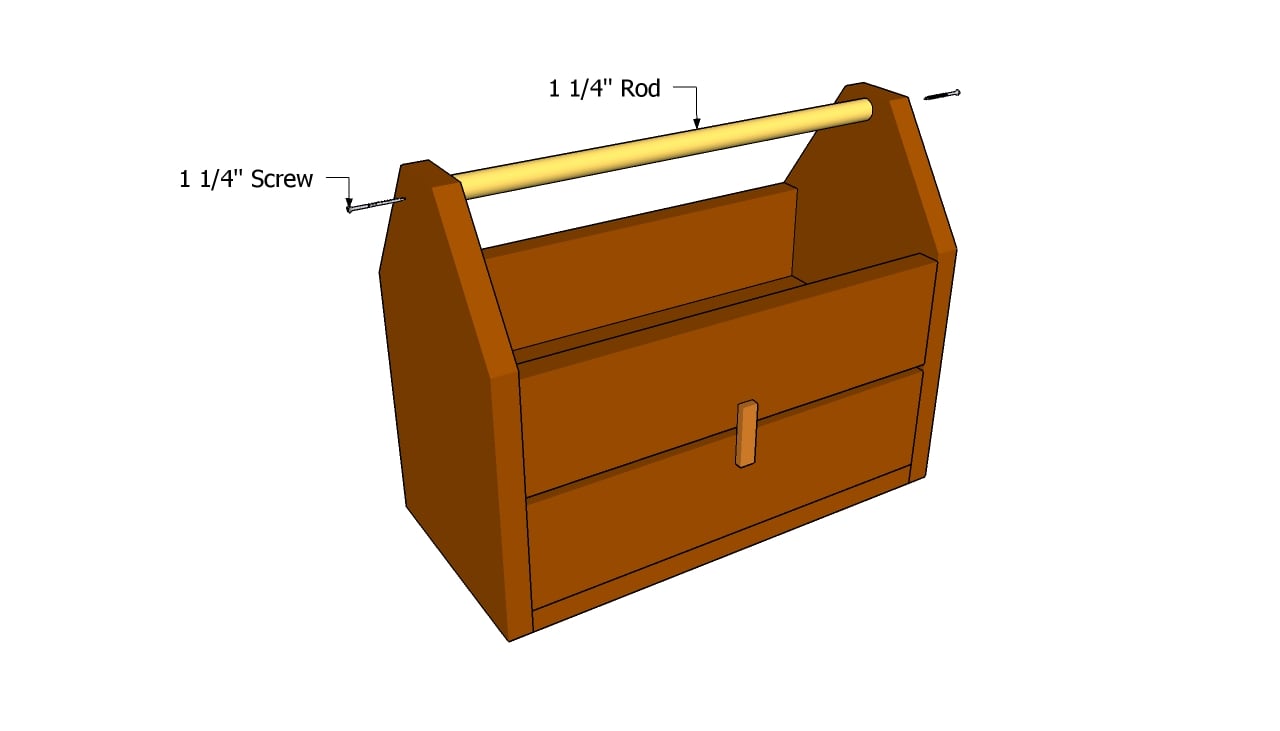The image depicted is a detailed cartoon diagram of a vintage wooden toolbox, typically used around the 1950s in contexts such as car repair or light building construction for quick access to tools. The toolbox itself is a light brown, double-open design with two distinct sections. The top section resembles a traditional open toolbox, and the lower section appears to have a latch closure. A prominent feature is a yellow rod handle on the top, which is secured by screws on each side. Specifically, the screws are designated as one and one quarter inch in size, as indicated by labels pointing to their locations on each side of the rod. This information highlights how the handle is attached to the sturdy wooden structure.